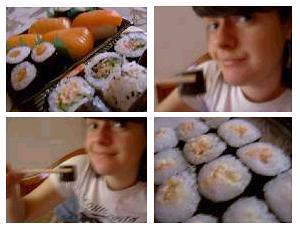The image is a collage consisting of four neatly arranged photographs, resembling a window pane with two pictures on the top and two on the bottom. The top-left section showcases an assortment of sushi rolls accompanied by sashimi. The top-right photo captures a close-up of a smiling woman holding a piece of sushi with tan brown or beige chopsticks, poised as if about to eat it while looking at the camera. The bottom-left image features the same woman holding the sushi in a similar manner, with the piece slightly moved, as if she is bringing it toward her mouth but still smiling at the camera. Finally, the bottom-right photograph provides a closer view of the sushi, highlighting the intricate details of the sushi rolls on a tray.